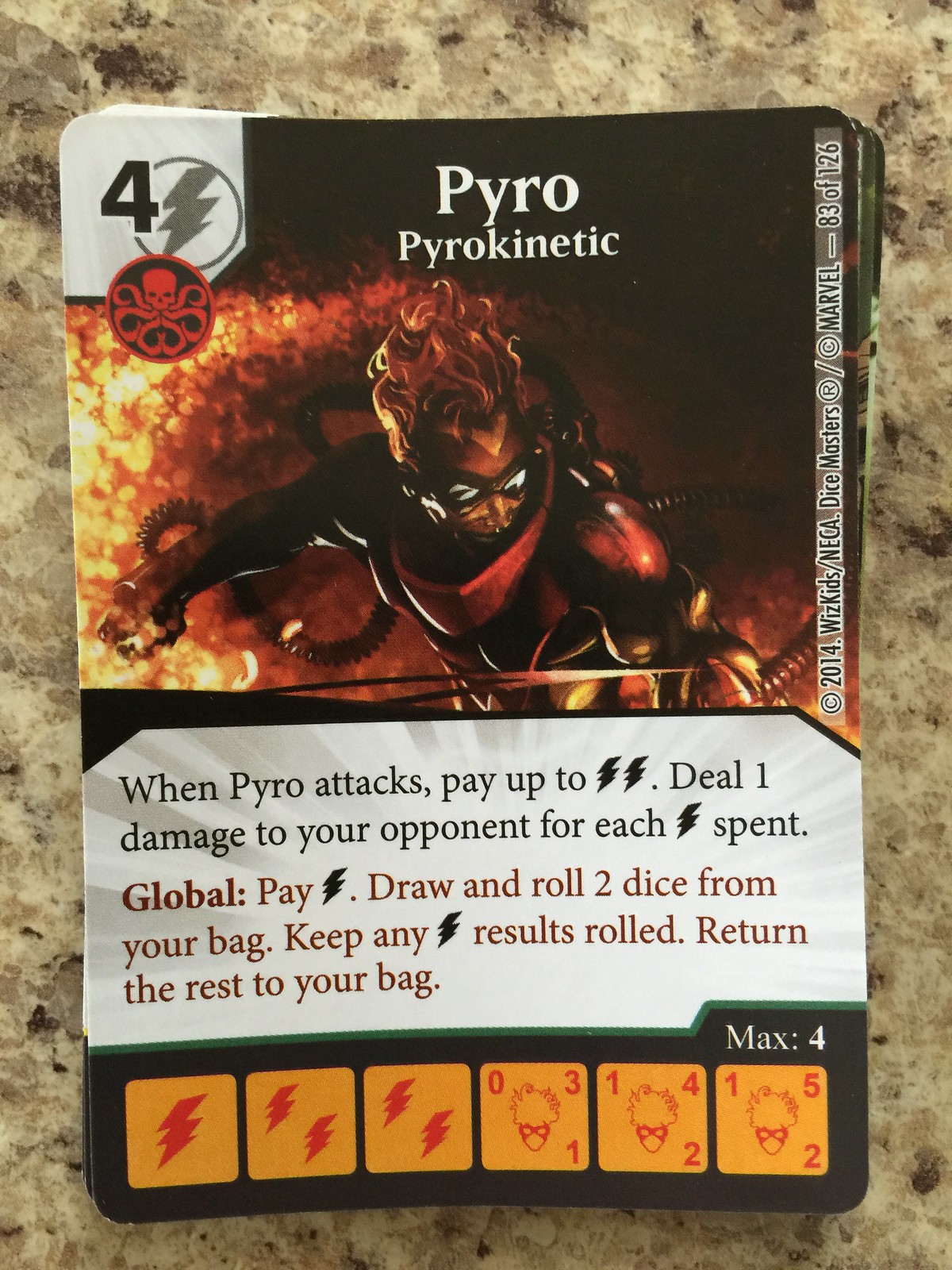On a gray sandstone surface lies a collection of trading cards, the top one prominently featuring a superhero named Pyro in a bold, red suit. This character has fiery red hair, and flames emanate from his hand, enhancing his menacing demonic appearance. Particularly eye-catching are the pipes incorporated into his suit, adding to his intricate design. In the upper left corner of the card, the number "4" is displayed next to a lightning bolt icon, indicating its power level. The top of the card reads "Pyro" and "Pyrokinetic" in white text against a dark backdrop.

The card is meticulously detailed: on the upper right corner, it indicates it's part of a collection with "83 of 126," and a visible copyright notice states "2014 WizKids Mega Dice Masters Marvel." The card also contains specific gameplay instructions. Printed in white, it reads: "When Pyro attacks, pay up to two lightning bolts to deal one damage to your opponent for each lightning bolt spent. Global: Pay one lightning bolt to draw and roll two dice from your bag. Keep any lightning bolt results rolled; return the rest to your bag." At the bottom, there are small, orange rounded squares with lightning bolt icons and facial images of the character, adding to the card's elaborate design.